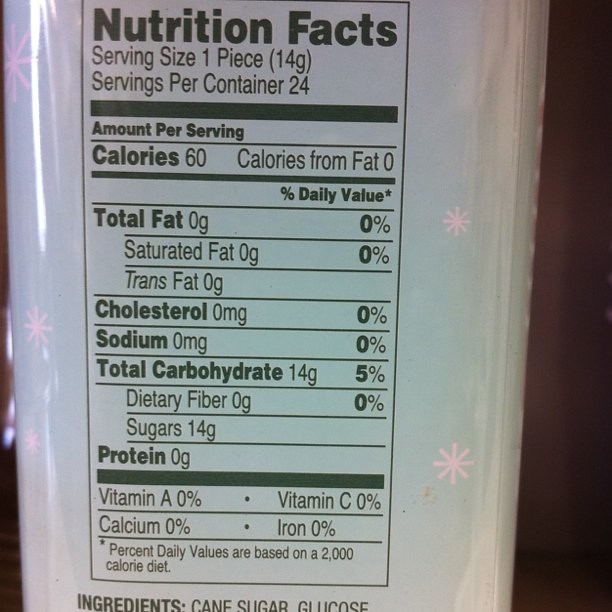This image features a detailed Nutrition Facts label displayed on the side of a clear plastic box. The label, printed in black ink on a crisp white background, provides the following information:

- **Serving size:** 1 piece (14 grams)
- **Servings per container:** 24
- **Calories:** 60
- **Calories from fat:** 0
- **Total fat:** 0 grams (0% Daily Value)
- **Saturated fat:** 0 grams (0% Daily Value)
- **Trans fat:** 0 grams (0% Daily Value)
- **Cholesterol:** 0 milligrams (0% Daily Value)
- **Sodium:** 0 milligrams (0% Daily Value)
- **Total carbohydrates:** 14 grams (5% Daily Value)
- **Dietary fiber:** 0 grams
- **Sugars:** 14 grams

The primary ingredients listed are cane sugar and glucose, indicating that the product consists mostly of sugar.